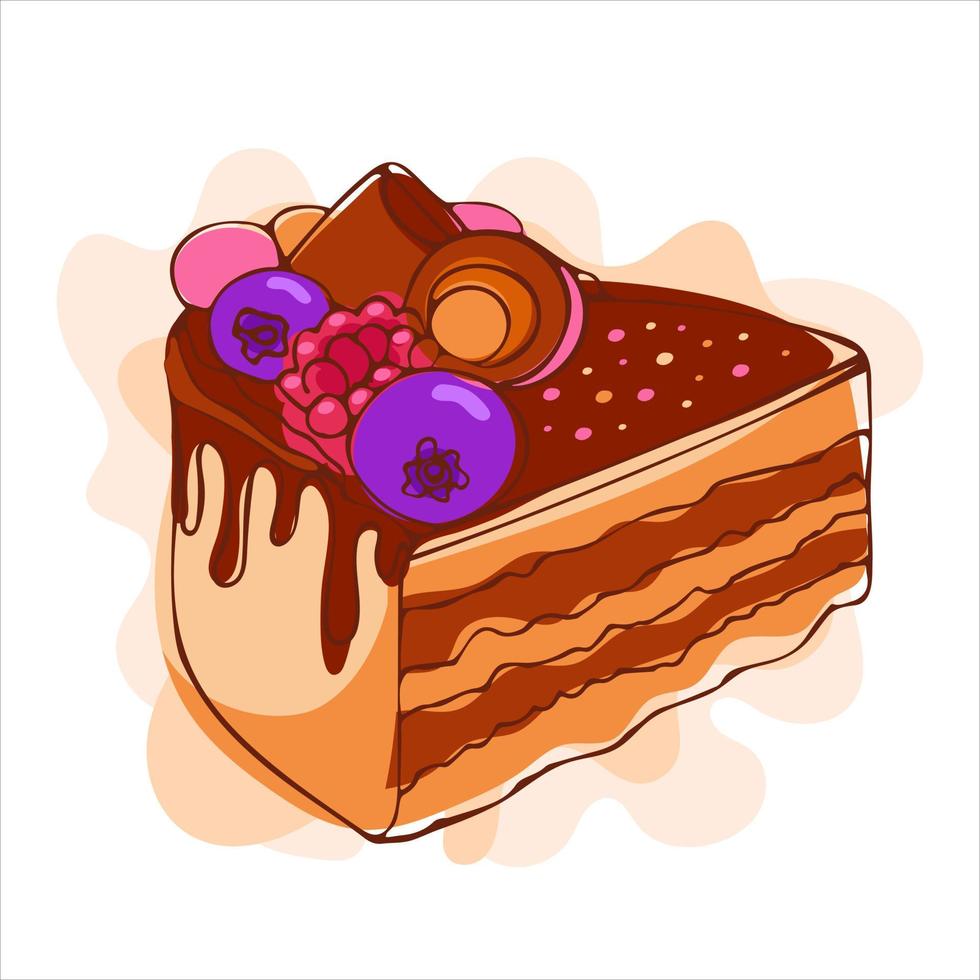The illustration is a detailed clipart of a slice of layered cake set against a bright white background with irregular beige and orange splotches. The cake slice is presented with the cut portion slightly facing to the right, revealing its intricately alternating orange and brown wavy layers, each bordered with brown outlines. The curved exterior edge on the left side is accented by a beige circle and an orange crescent. Brown frosting drips down one side, covering the top and adorned with an assortment of colorful decorations. On the right end, there are pink, orange, and white dotted sprinkles. On the left, two large purple berries, likely grapes, flank a pink flower. Further to the right, two pieces of brown chocolate nestle among the decorations. The illustration's colors are slightly offset, giving it a whimsical and lively appearance.